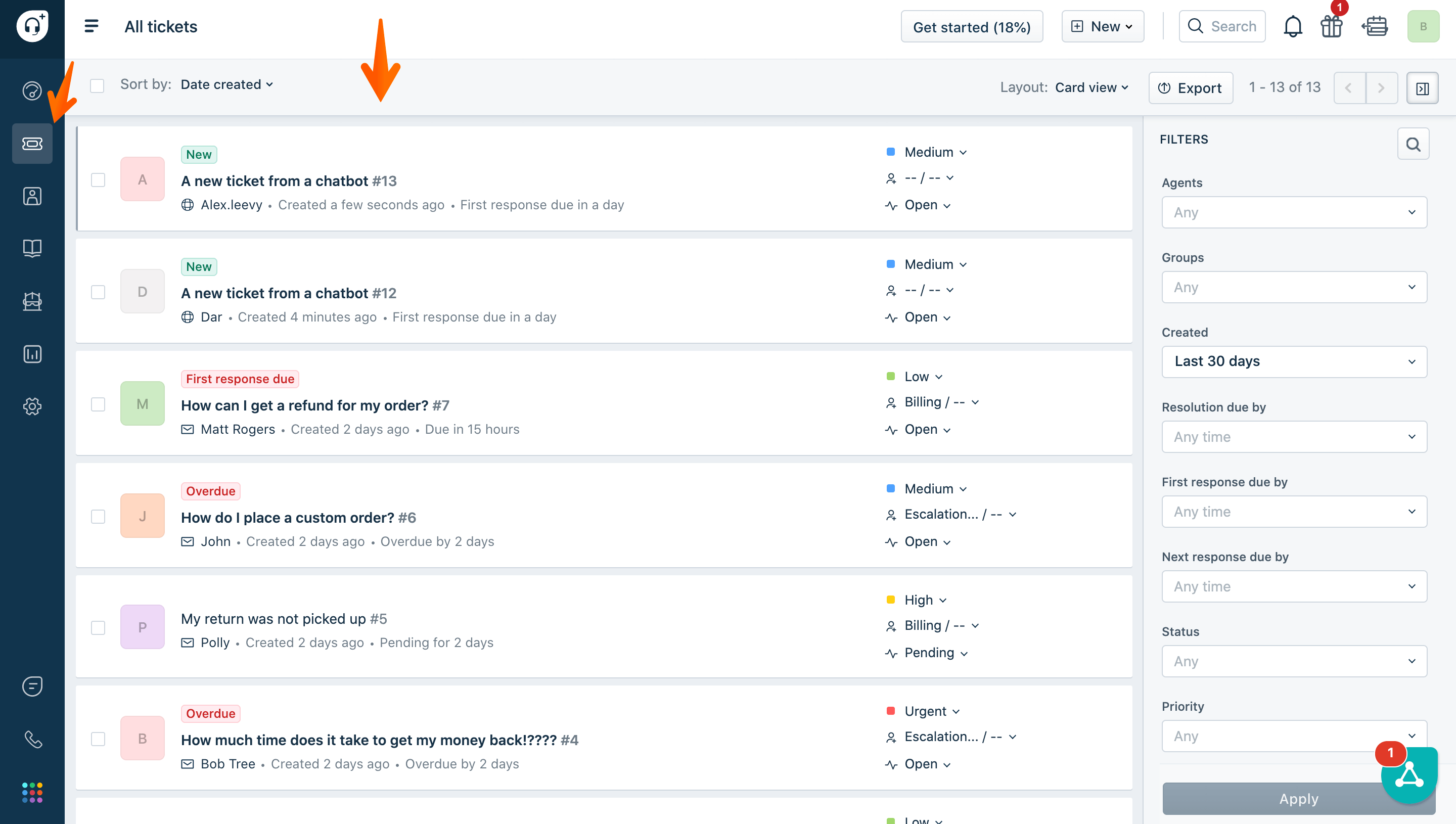The image portrays a detailed customer support dashboard interface, highlighting a ticket management system. At the top, there is a navigation bar that includes an "All Tickets" dropdown with a context menu, a "Get Started" progress indicator at 18%, a search function, and icons for gifts and notifications, along with a save button.

On the left-hand side, a vertical blue bar contains menu options—though slightly unclear, it appears to include icons representing tickets, profiles, graphs, and settings.

The main section of the dashboard displays ticket listings sorted by creation date with various urgency levels marked. The first ticket, labeled "New Ticket from Chatbot 13" with medium urgency, is followed by "New Ticket from Chatbot 12," also marked medium and currently open. Subsequent tickets include:
- "First response to: 'How do I get the refund for my order number seven'" by Matt Rogers, indicating it is overdue.
- "How to place a custom order number six" by John, created two days ago and overdue.
- "My return was not picked up, number five" by Polly, created two days ago, pending for two days, and overdue.
- "How much time does it take to get my money back, number four," marked as urgent.
- Another high-priority ticket is also listed last.

On the right side of the interface, there are additional options and search functionalities to further filter and manage the tickets, providing a comprehensive tool for tech support and customer service management.